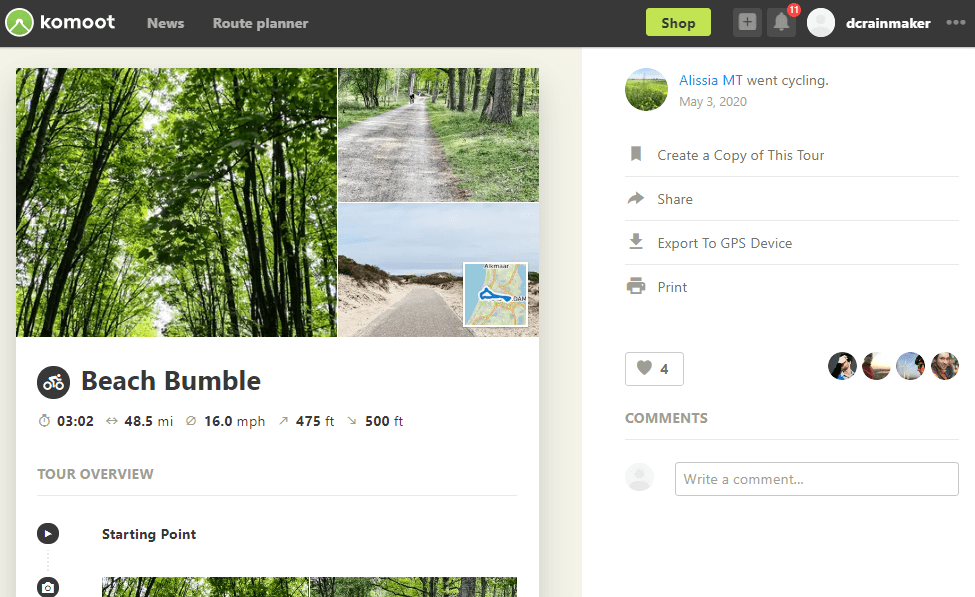This image captures a screenshot from the Kormoot website. Dominating the top of the webpage is a dark gray, nearly black, border. Situated in the upper left corner, the company name "Kormoot" is prominently displayed in bold, white, lowercase letters. Accompanying this is a green circle housing a white, stylized mountain peak.

To the right of the company logo, the menu items "News" and "Route Planner" are presented in a light gray font. On the far right of the top border, a green rectangle bearing the word "Shop" in black font stands out. Adjacent to this is a gray square featuring a dark gray plus sign, followed by a gray notification bell marked by a red circle with the white number "11," indicating 11 notifications. The user's name, "DCRainmaker," is shown in gray font, all lowercase and run together.

The upper left section features a photo of trees with lush green leaves and narrow, dark gray tree trunks. Below this, a second image displays an unpaved dirt path surrounded by green grass and tree trunks. In the lower right corner, another photo depicts a one-lane road set in a desert-like, arid landscape with distant mountains under a hazy blue sky.

Below these images, against a white background, the text "Beach Bumble" is displayed, followed by "Tour Overview" in gray font, and then "Starting Point," indicating further details about the tour that are not visible in this screenshot.